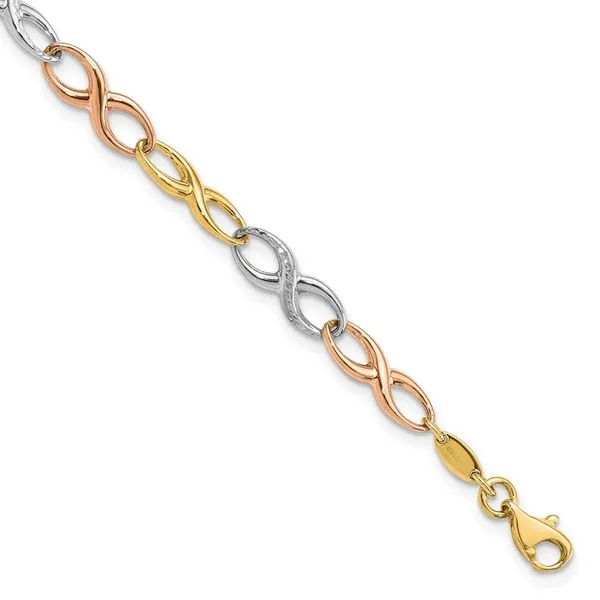The image showcases a delicate and shiny bracelet photographed against a white background, running diagonally from the top-left (northwest) to the bottom-right (southeast) of the frame. The bracelet features an intricate double helix design interspersed with figure-eight links made of gold, rose gold, and silver. Starting at the top-left, a silver fastener initiates the bracelet, followed by a rose gold figure-eight link, then a silver figure-eight link adorned with a central design resembling tiny diamonds. This sequence continues with a regular gold figure-eight link and another rose gold figure-eight link. The bottom-right end of the bracelet terminates with a gold link connected to a clasp that includes a pull-down pin for opening. This elegant piece intertwines varying metallic hues in a sophisticated pattern, exuding a sense of delicate craftsmanship.